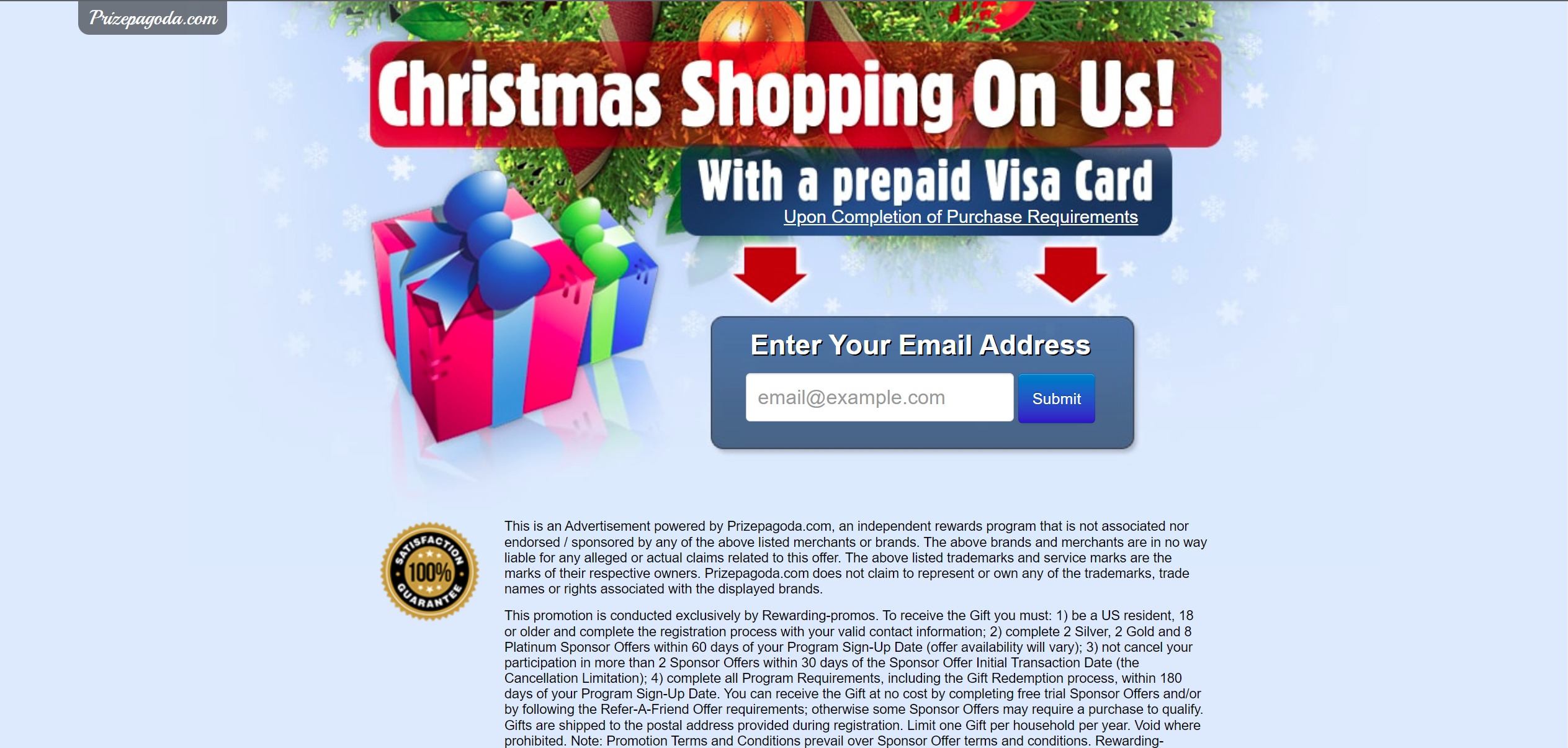Horizontal screenshot of a promotional webpage from PrizePagoda.com, featuring a holiday-themed advertisement. The top part of the screenshot is dominated by a red banner overlaid on a background of a Christmas tree decorated with ornaments. The banner reads "Christmas Shopping on Us" in white text, followed by a dark blue bubble with the text "with a prepaid VISA card." Below this, a link states "upon completion of purchase requirements." Flanking the text are two cartoon gift packages. Beneath this section are two large red arrows pointing downwards towards a blue box. This box contains the text "Enter your email address," accompanied by a white text box for email submission and a "Submit" button. In the lower left quadrant, there's a seal that says "100% Guarantee" in white, black, and gold. Adjacent to the seal are two paragraphs of fine print, with the first paragraph beginning, "This is an advertisement powered by PrizePagoda.com, an independent rewards program that is not associated," and the second paragraph starting with, "This promotion is conducted exclusively by Rewarding Promos. To receive the gift you must," followed by a list of conditions for receiving the gift. The overall color scheme and festive visuals emphasize the Christmas theme of the advertisement.